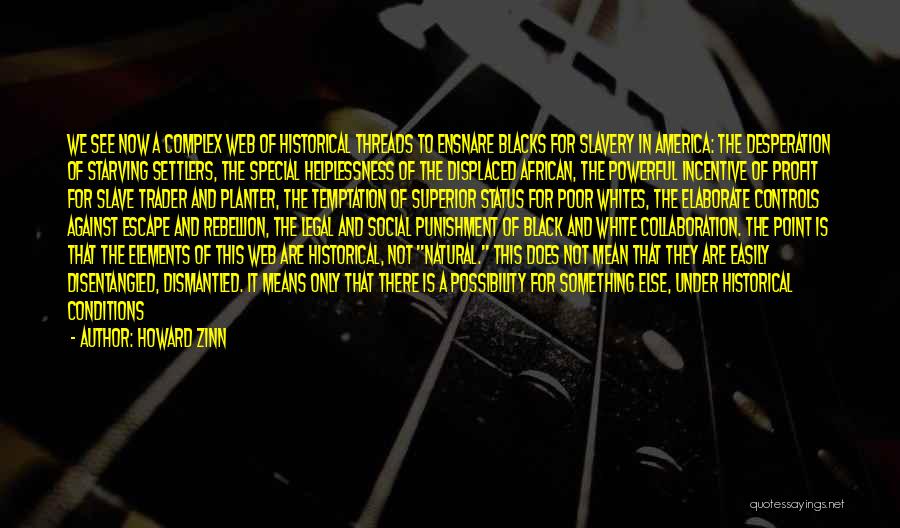The image features a quote by Howard Zinn in bold yellow text on a dark background with white patterns that resemble the blurred strings of an electric guitar facing down and slightly to the left. The detailed quote discusses the complex historical web of factors that contributed to the enslavement of blacks in America, including the desperation of starving settlers, the helplessness of displaced Africans, the profit incentives for slave traders and planters, the temptation of superior status for poor whites, the elaborate controls against escape and rebellion, and the legal and social punishment of black and white collaboration. The quote emphasizes that these elements are historical, not "natural," suggesting that while they are not easily dismantled, there is a possibility for change under historical conditions. The text concludes with "author: Howard Zinn" and in the bottom right corner, the small light gray text reads quotesayings.net.